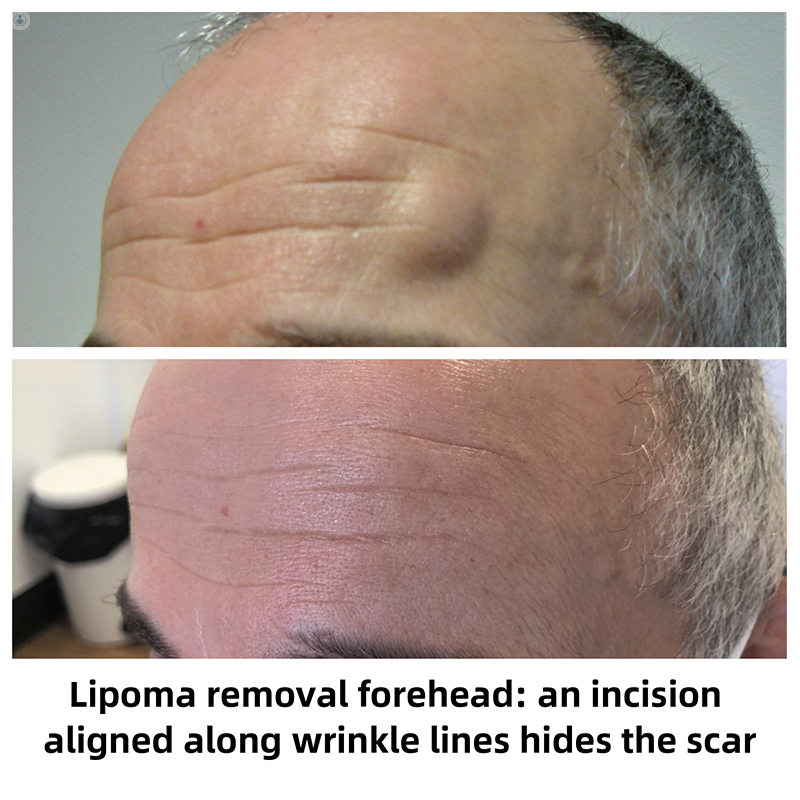This is an informative composite image comparing the forehead of a Caucasian male before and after lipoma removal. The photo set features two landscape-oriented photographs. The top image shows the man's forehead where several pronounced lumps, or lipomas, are visible, accentuating his wrinkles. He appears to be in his 50s or early 60s, with thinning, graying hair mostly on the sides of his head. The second image, located beneath the first, illustrates the same man's forehead post-removal. Here, the lumps have been effectively eliminated, and only the natural wrinkles remain, seamlessly camouflaging the surgical scars thanks to an incision technique aligned with the wrinkles. The text below the images reads: "Lipoma removal forehead: An incision aligned along wrinkle lines hides the scar," emphasizing the surgical approach taken to ensure minimal visible scarring. The background of the first image is a plain whitish-gray wall, while the second image includes additional elements like part of a wall and a garbage pail in the bottom left corner.